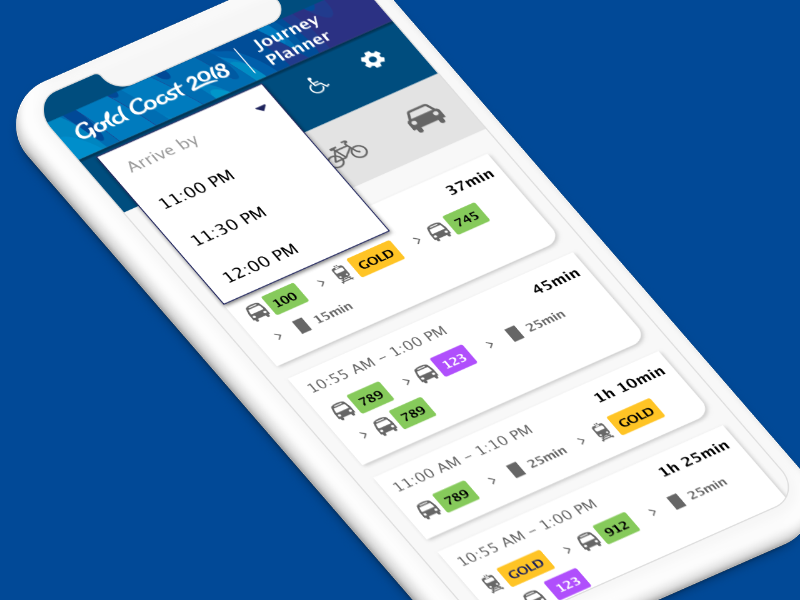A detailed descriptive caption for the image could be:

"The image features a blue rectangle with a longer horizontal dimension than vertical, serving as the backdrop. Positioned diagonally from the top left to the bottom right of the rectangle is a white smartphone displaying the 'Gold Coast 2018 Journey Planner' app. The screen of the smartphone shows a drop-down menu for selecting an arrival time with options like 11:00 PM, 11:30 PM, and 12:00 PM. Adjacent to the menu, there's a handicap symbol and a settings icon. Below this section, several transport options are represented with icons: a bicycle and a car on the right side.

Next to these icons, the text indicates a travel time of 37 minutes for some option. Further down, the screen suggests a route where 'Bus' is prominently mentioned with a numeric indicator, likely a route number, saying '100.' Following this, there's a section marked 'Gold' in yellow, next to another route option labeled '745 Bus.' An arrow pointing to the right suggests additional details or navigation.

At the bottom part of the phone's screen, the image shows scheduled times, like 10:55 AM through 1:00 PM, with varying travel durations. For instance, '45 minutes' for one segment, and 'Bus 789' or 'Bus 1 2 3' options with times like '25 minutes' and others. It also includes repeated details about the 'Train or Bus 789' options.

All these details are laid out in an easy-to-follow format, making the journey planning process efficient and accessible."